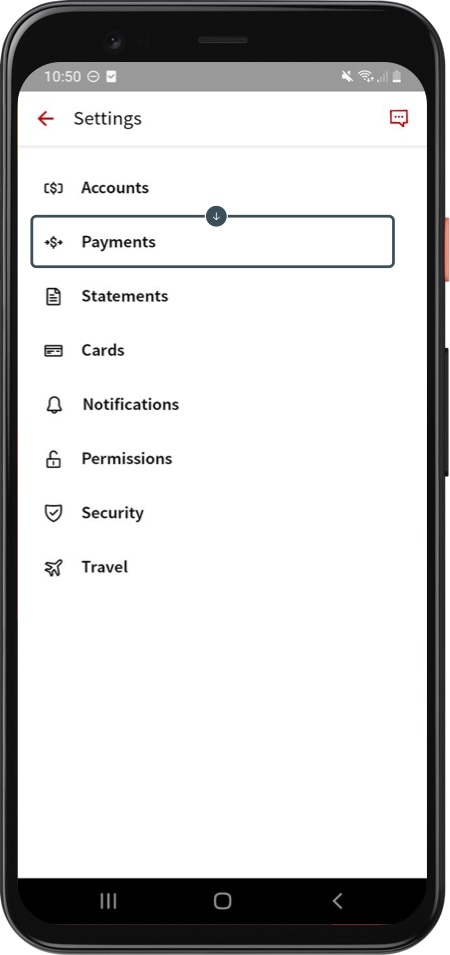In this detailed image of a cell phone screen set against a gray background, a multitude of interface elements and icons are meticulously displayed.

The screen features a two-layered border, with an outer black edge and an inner brown edge. At the top of the brown section, the time "10:50" is prominently displayed in gray text. Nearby, several status icons are visible: a gray circle, a white square, and to the right, indicators for low battery power and weak Wi-Fi signal. Additionally, the volume icon indicates that the phone is on mute.

Moving downwards, the screen's main content begins. The first line contains a red arrow pointing to the left and the word "Settings" in bold black font. To the right of this is a square icon with three dots and a descending line.

A light gray line separates this section from the next. Here, you'll find an entry marked with square brackets enclosing a dollar sign, labelled "Accounts". Below this, there is an icon of a gray circle with a downward-pointing arrow, a dollar sign with two dots beside it, and the label "Payments".

The subsequent lines continue with similar detailed entries:
- A square icon with three lines, labelled "Statements".
- A square icon with two lines, labelled "Cards".
- A bell icon, labelled "Notifications".
- An open padlock icon, labelled "Permissions".
- A crest icon with a check mark inside, labelled "Security".
- An airplane icon, labelled "Travel".

At the very bottom of the screen, a black horizontal line is present, featuring three vertical lines of varying heights, a rounded square in the center, and an arrow pointing to the left.

This thorough representation highlights the intricate layout of the phone's user interface, with clear labeling and iconic imagery for easy navigation and user interaction.